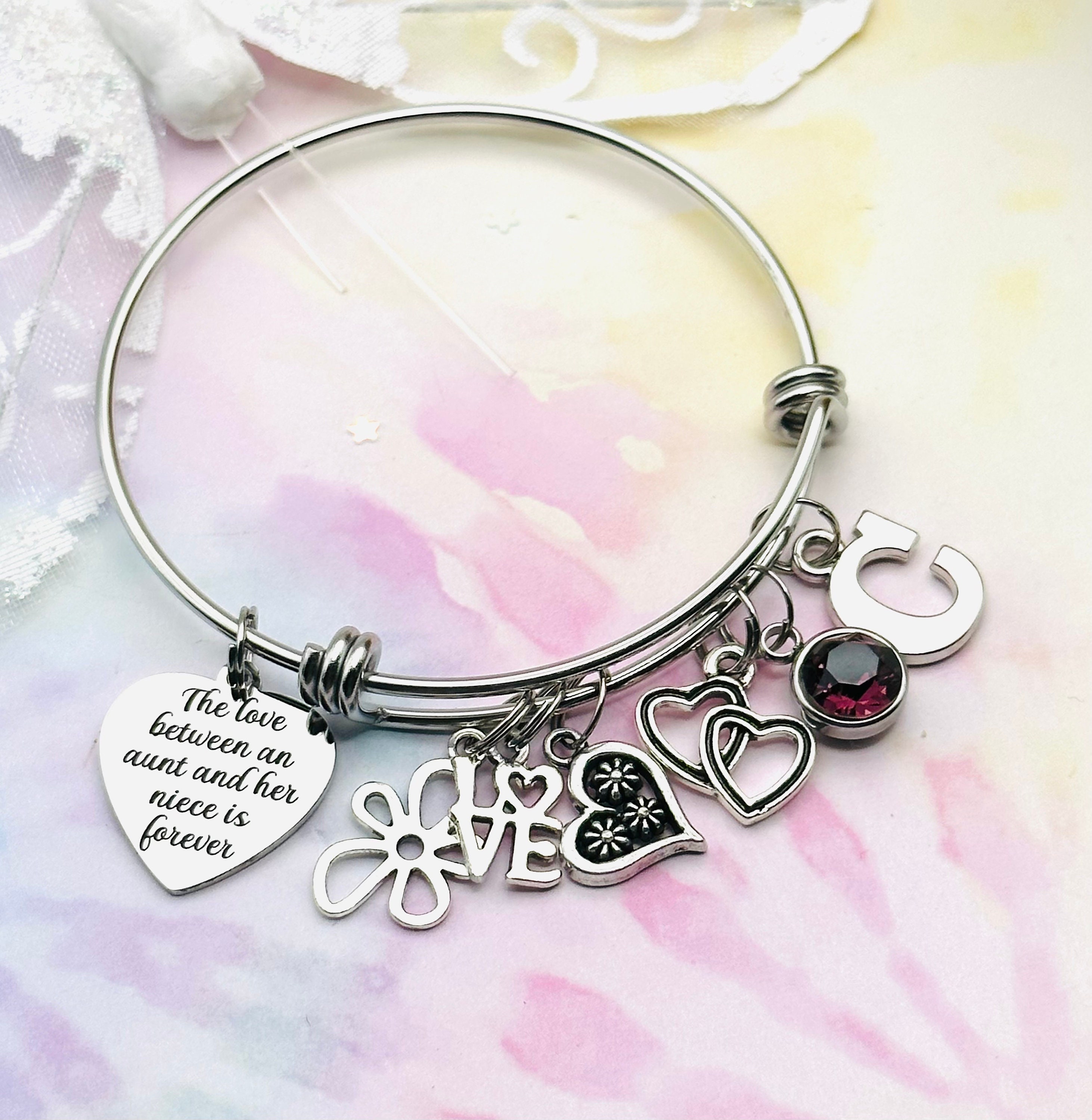The image features a delicate silver friendship bracelet adorned with a series of intricate charms. The bracelet is artistically laid on a muted pinkish-purple fabric with subtle hints of white lace in the upper left and right corners, adding a feminine touch to the scene. The bracelet itself is composed of thin wire, shimmering with a soft silver luster. From left to right, the charms include: a heart engraved with the heartfelt inscription, "The love between an aunt and her niece is forever;" a unique flower with petals of varying shapes and sizes; a square charm featuring the word "LOVE" with an innovative design where the O's are heart-shaped; another heart with delicate snowflake patterns; a pair of interlocked hollow hearts merging silver and black; a small round amethyst gemstone set in silver; and finally, a silver letter "C". This carefully arranged composition highlights the sentimental value and elegance of the bracelet.